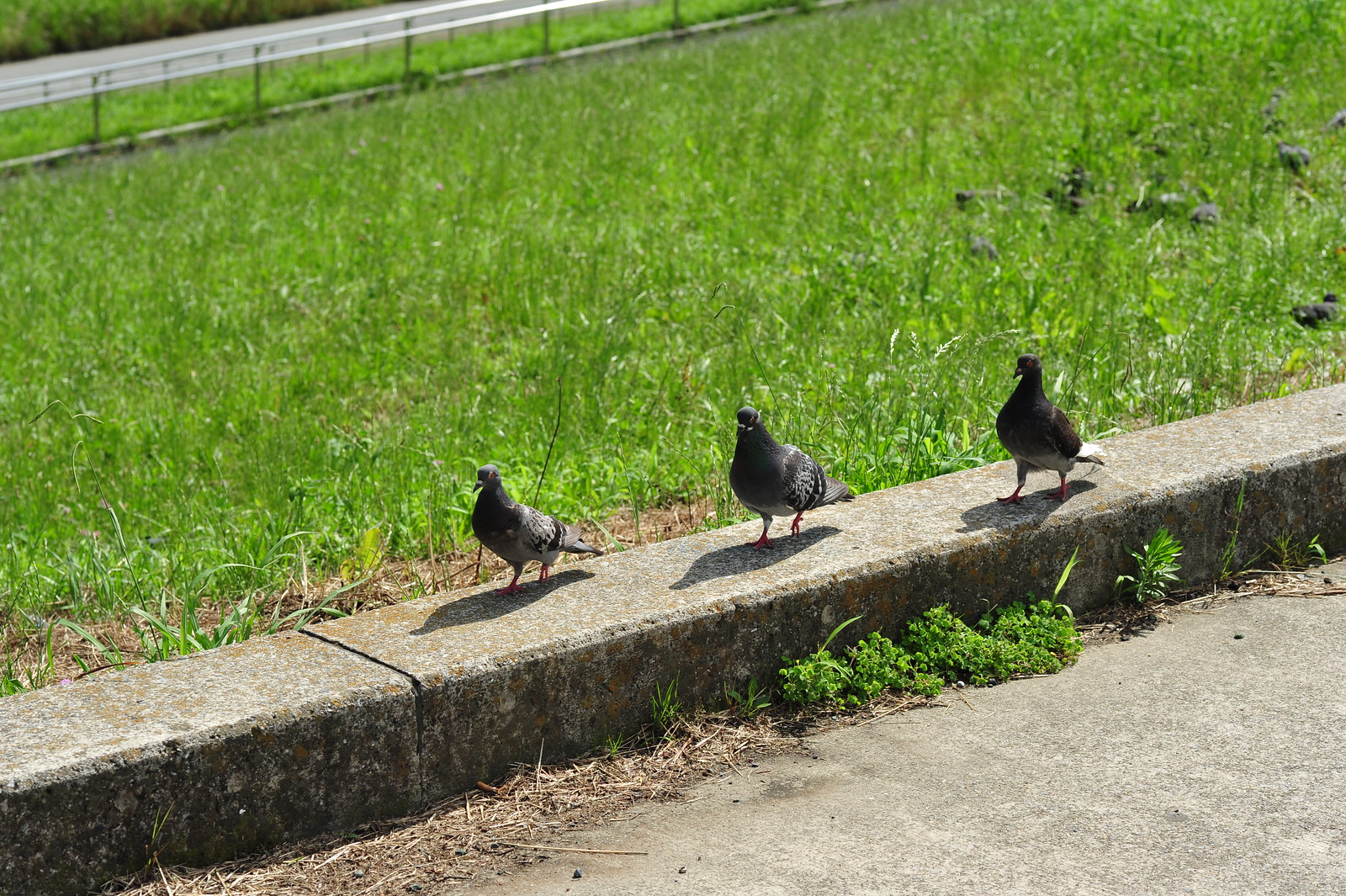The photograph captures three gray pigeons with black markings and orange legs, walking along a broad, flat concrete curb that runs diagonally from the top right to the bottom left of the image. The birds are spaced evenly and moving in the same direction, providing a clear profile view. At the junction of the curb and the sidewalk in the foreground, green weeds are sprouting amidst debris of dirt and old grass. On one side of the curb lies a cement sidewalk, while on the other side is a patch of long, tall green grass. The background features a silver fence that resembles aluminum bleachers, adding an element of ambiguity as it flanks what appears to be a single-lane road. The photograph, taken in color and from an elevated angle, presents an outdoor scene combining urban and natural elements.